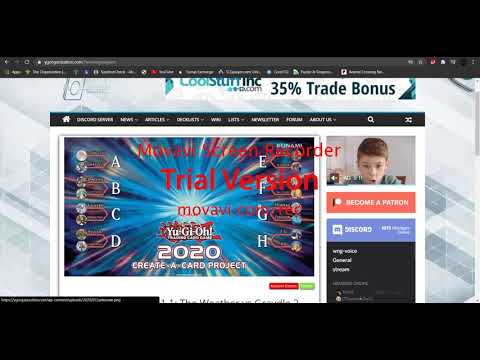The image is a detailed screenshot of a web browser, likely Chrome, displaying a website with a somewhat dated and sketchy appearance. The browser has a black-themed style with various tabs and bookmarks visible. On the web page itself, there's a prominent banner advertisement for CoolStuffInc.com offering a "35% trade bonus," displayed in blue. The primary content of the site features material related to Yu-Gi-Oh!, specifically a "2020 Create-A-Card Project," surrounded by a dramatic graphic design with blue lines converging into a bright center. 

At the top and bottom of the screenshot, there are black rectangles stretching from left to right, indicating the area captured by the screen recording software. Notably, a red watermark indicates that a Movavi screen recorder trial version was used, with "trial version" emphasized in a larger font. In the upper right section of the web page, there's an image of a child with brown hair and an 'O' shaped mouth, giving a surprised reaction to the content. Below this image, there's a salmon-colored button labeled "Become a Patron," encouraging viewers to support the content creator. Additional elements on the page include links to a Discord and other related information about the Yu-Gi-Oh! project. Overall, the site has an older aesthetic with patterned blue and white diagonal lines reminiscent of early web design, akin to MySpace.